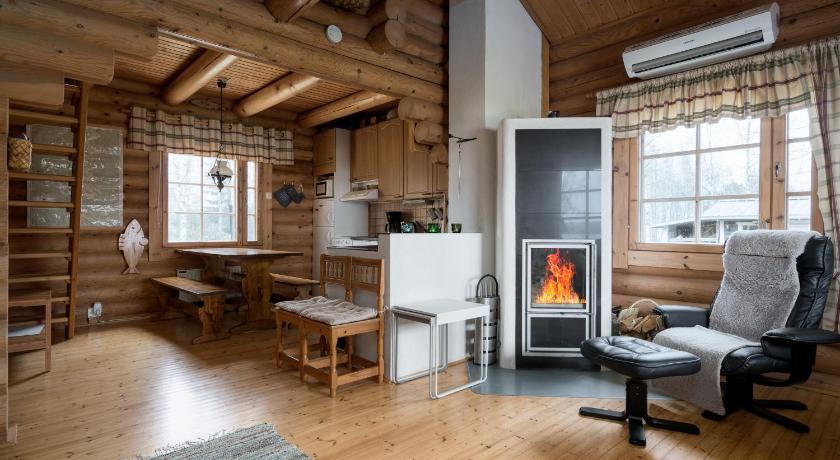In this color photograph of a meticulously kept log cabin interior, a warm, inviting, and distinctly rustic ambiance is captured. The scene is dominated by wooden elements, with polished wooden floors, walls made of logs, and a wood-beamed ceiling all contributing to the authentic cabin feel. 

In the foreground, at the bottom right, sits a tan leather easy chair paired with a black ottoman, both covered in a soft sheepskin, adding a cozy touch. To the left of the chair, a sleek, modern fireplace with a glass front and a white frame adds a contemporary twist to the otherwise rustic setting. Adjacent to the fireplace is a small kitchen area featuring a wood table with benches, surrounded by various wooden cabinets.

The room features a gray area rug in the bottom left corner and includes several functional elements such as an air conditioner and a refrigerator, ensuring comfort. Decorative touches like fish ornaments hanging on the logs add charm and personality. Two windows with white curtains embellished with green and red stripes provide natural light, flanking either side of the room. In the middle, two wooden chairs with white upholstered pads complement the setting. 

A wooden ladder indicates access to another level of the home, hinting at a multi-functional space. The overall palette includes shades of brown, gray, black, red, yellow, and white, bringing cohesion and warmth to this log cabin interior.